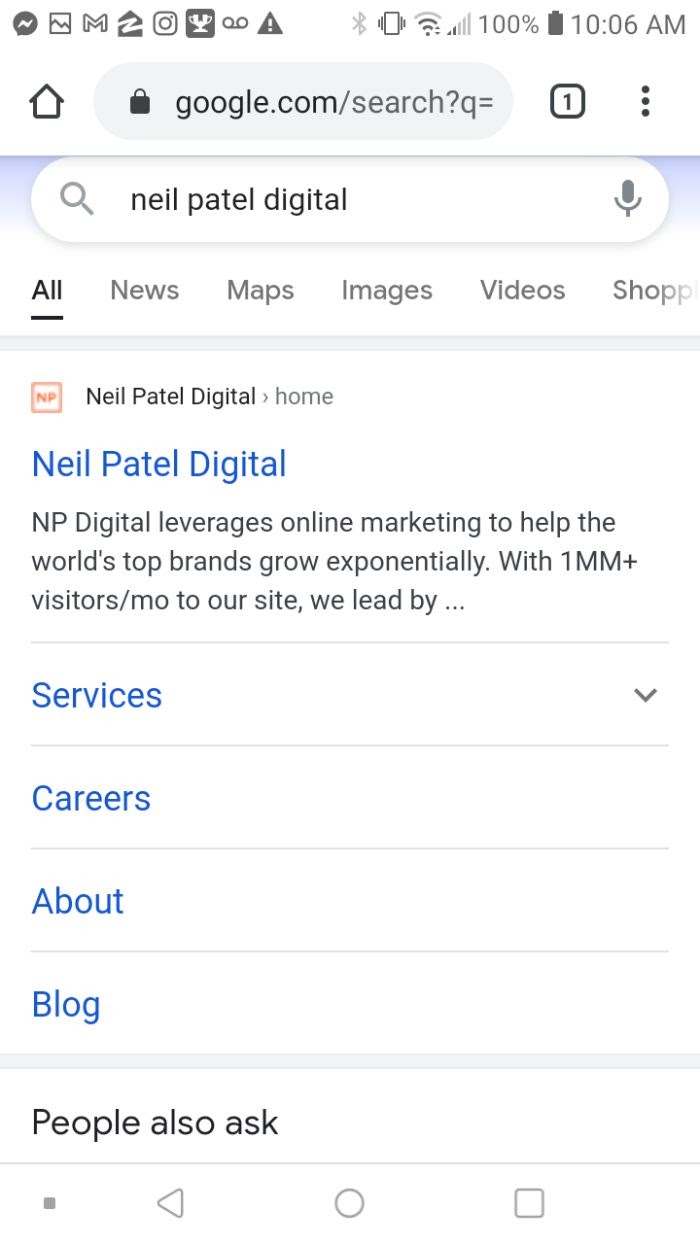The image is a detailed screenshot captured from a mobile device, showcasing various elements typical of a smartphone interface. Along the top of the screen, a dense array of notification icons is visible, indicating activities from multiple applications on the left-hand side. On the right-hand side, the status bar displays icons for Bluetooth connectivity, Wi-Fi connection, network signal strength, battery status, and the current time.

Centered below the status bar, the browser window is open to a Google search page. The search bar indicates the active query, "Neil Patel Digital," with the results of the search displayed underneath. The lone search result features a link to the Neil Patel Digital website, accompanied by quick navigation hyperlinks to sections like Services, Careers, About, and Blog.

At the bottom of the screen, the standard navigational buttons for the mobile device are present: a backward-facing triangle for returning to the previous screen, a circle for going to the home screen, and a square for accessing recently used applications.